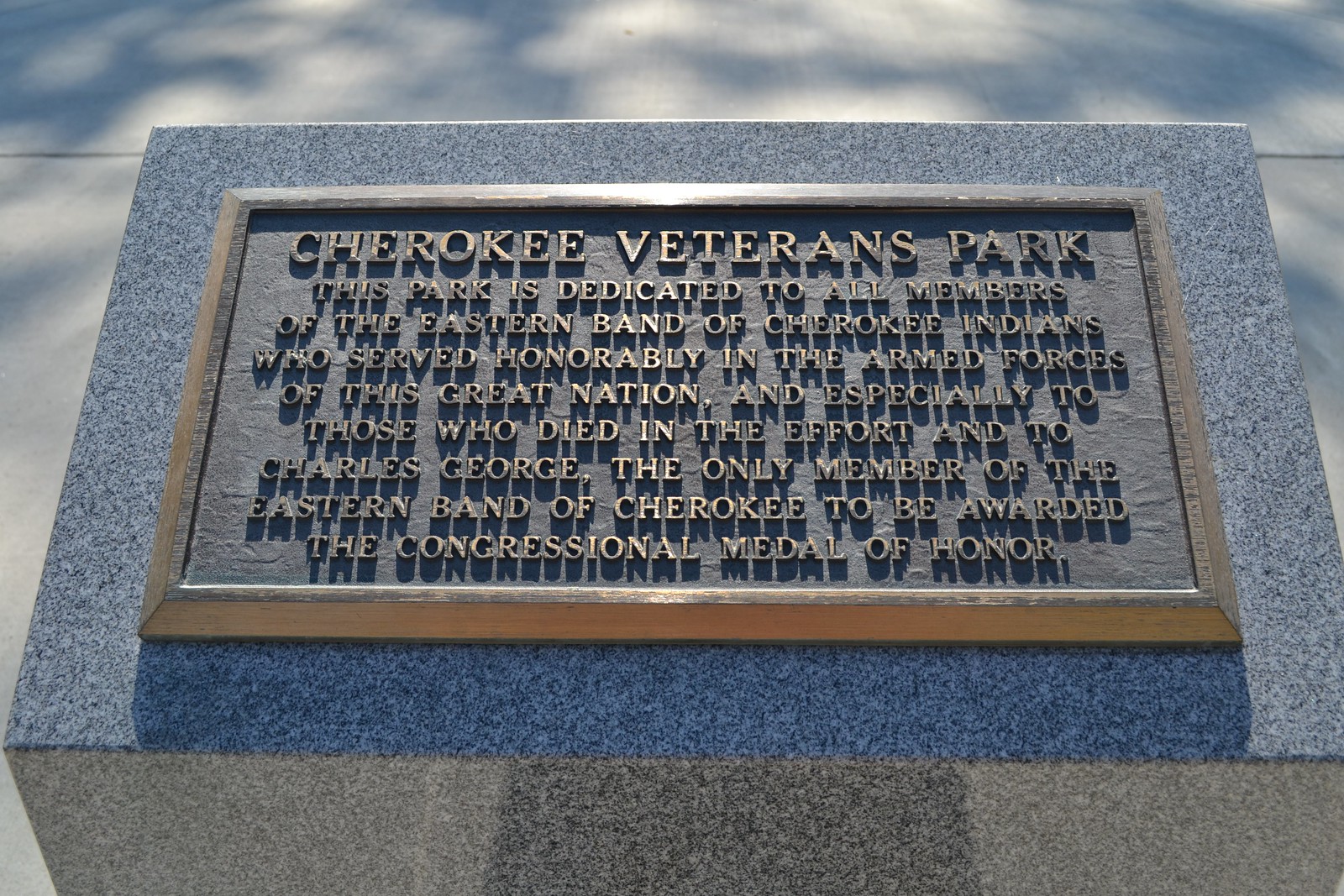The image depicts a horizontal, square monument constructed from granite or marble. This stone has a polished gray surface flecked with darker grays, blacks, and occasional white specks. Attached to the monument is a metal plaque with a brassy, raised gold border. At the top, it prominently reads "Cherokee Veterans Park." Below this title, the plaque bears an inscription: "This park is dedicated to all members of the Eastern Band of Cherokee Indians who served honorably in the armed forces of this great nation, and especially to those who died in the effort, and to Charles George, the only member of the Eastern Band of Cherokee to be awarded the Congressional Medal of Honor." The monument, situated outdoors on a cement ground, serves as a tribute to the Cherokee veterans, honoring their service and sacrifices in the military.